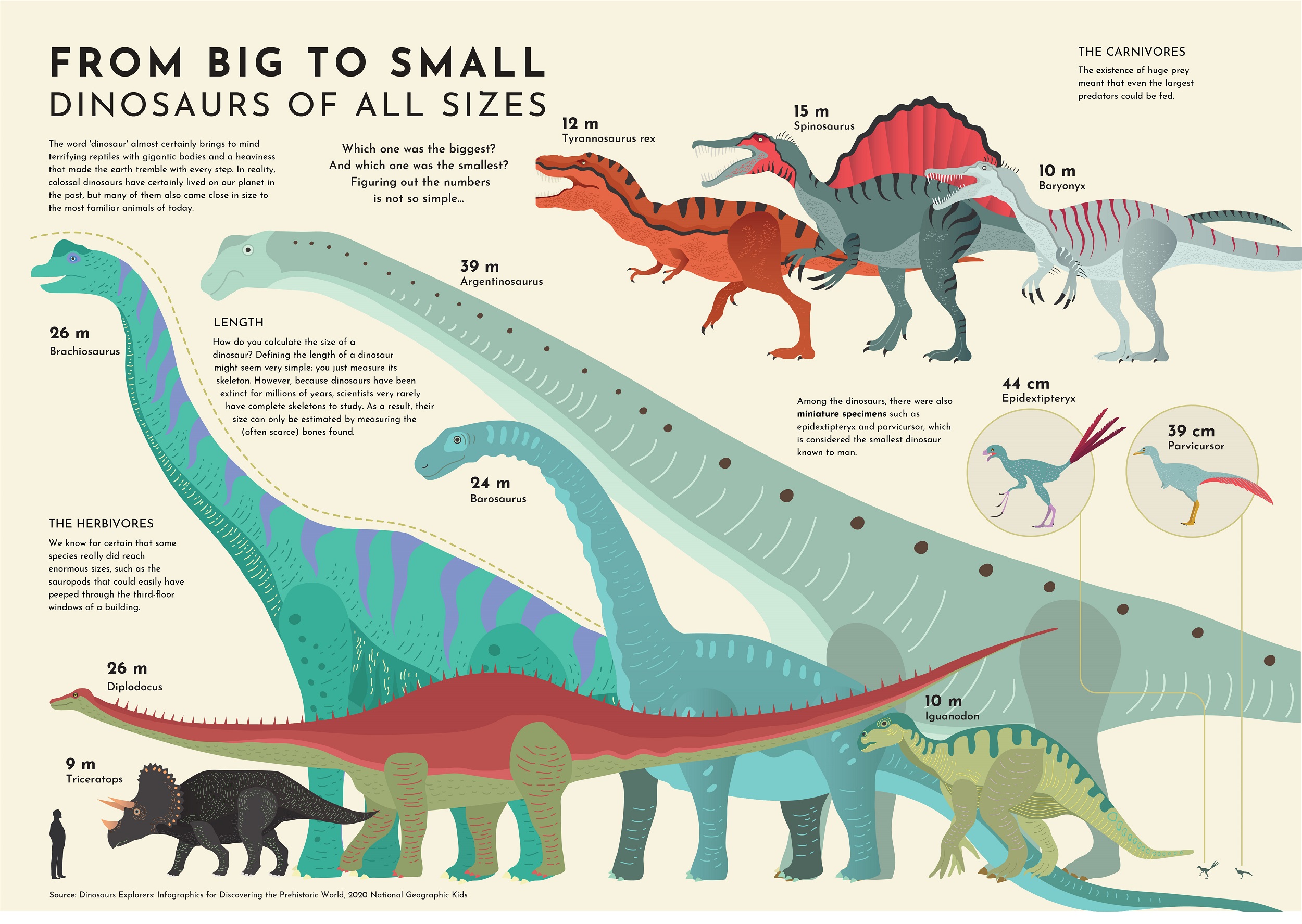This image is a comprehensive chart showcasing the size variations among different dinosaurs. Entitled "From Big to Small Dinosaurs of All Sizes" in a sans serif font, the chart features a white background filled with a multitude of dinosaur illustrations in various colors. Dominating the center is the largest dinosaur, an Argentinosaurus, measuring 39 meters in length. Nearby, the Brachiosaurus stands at 26 meters. 

The dinosaurs are depicted in an array of hues, including an orange Tyrannosaurus (12 meters) with small arms, and various other creatures in green, blue, red, and purple combinations. Notably, there is a green dinosaur with purple stripes and a red-topped, green-bottomed dinosaur with spikes. Additionally, a rhinoceros-like dinosaur adorned with a crown-like structure is also displayed. 

In the top left corner, a trio of dinosaurs with short forearms, long teeth, and beak-like snouts are positioned next to the title. Small text throughout the image poses questions such as "Which one was the biggest?" and "Which one was the smallest?" although much of it is too small to read. A human figure at the bottom left provides a scale reference to emphasize the enormous sizes of these prehistoric creatures. The background features subtle yellowish-green shading, adding depth to the visual presentation.